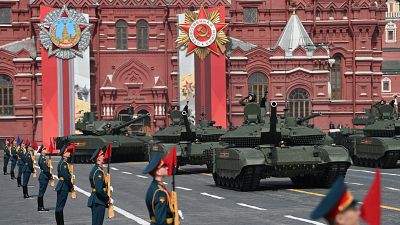The image captures a professional photograph taken during a daytime military parade in front of a significant dark maroon building, adorned with prominent emblems and banners. The focal point is the building, which features a large emblem above its entrance—on the left, a gold hammer and sickle mounted on a red circle and star, embellished with gold leaf and hanging banners. Another less discernible emblem on the right side also incorporates a red star, its details largely obscured by the emblem on top of it.

In the foreground, eight soldiers in blue military uniforms with yellow-gold trim stand in a disciplined formation. Each holds a rifle or a flag with red at the top, and they gaze straight ahead, facing the road. Along the street, three green tanks are visible in the middle, driving in a straight line, with an additional tank farther right in the background. The scene exudes a sense of order and formality, highlighted by the soldiers' stiff postures and the precision of the military vehicles. The entire scene, devoid of civilians, emphasizes a structured display of military presence.